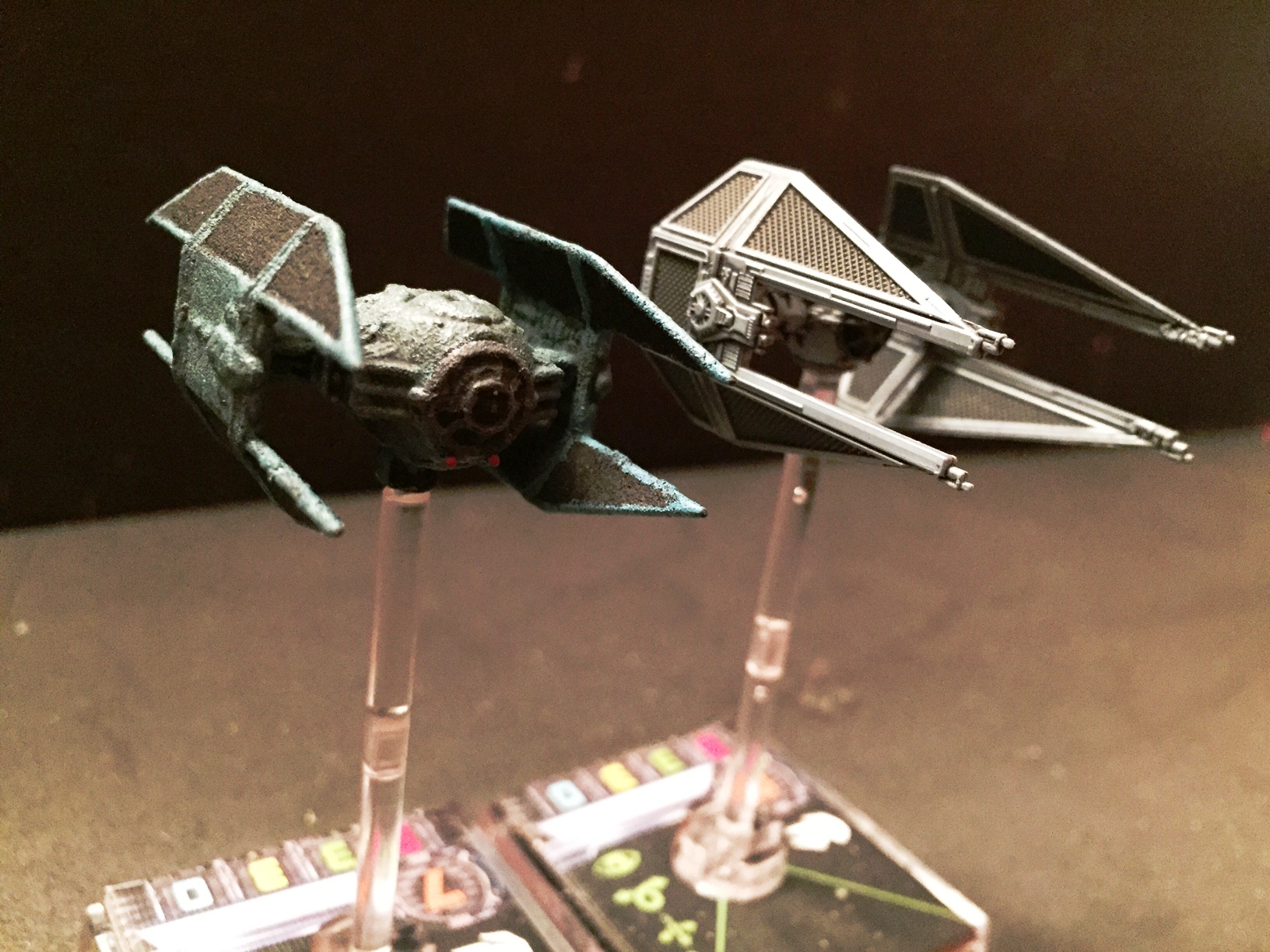This detailed color photograph, captured in a landscape orientation, showcases two small-scale replicas of TIE fighters from the Star Wars franchise, suspended on vertical clear plastic rods fixed into rectangular black bases adorned with intricate designs in white, green, red, and blue, reminiscent of sci-fi aesthetics. Both models are set on a gray table against a plain black backdrop. The left replica exhibits a chiseled, silvery blue central body with rounded wings that feature an intricate structure composed of triangular and square sections pointing upwards and downwards. Its central part has an octagonal front with a small circular window. The right-hand model features long, silvery wings with pointed ends, and although its central body isn't fully visible from the current perspective, the wings appear wider at the base and taper off distinctly. The bases of the mounts hold alien symbols, enhancing the otherworldly theme of the display. This representationally realistic image beautifully captures the intricate details and craftsmanship of these collectible Star Wars spacecraft models.